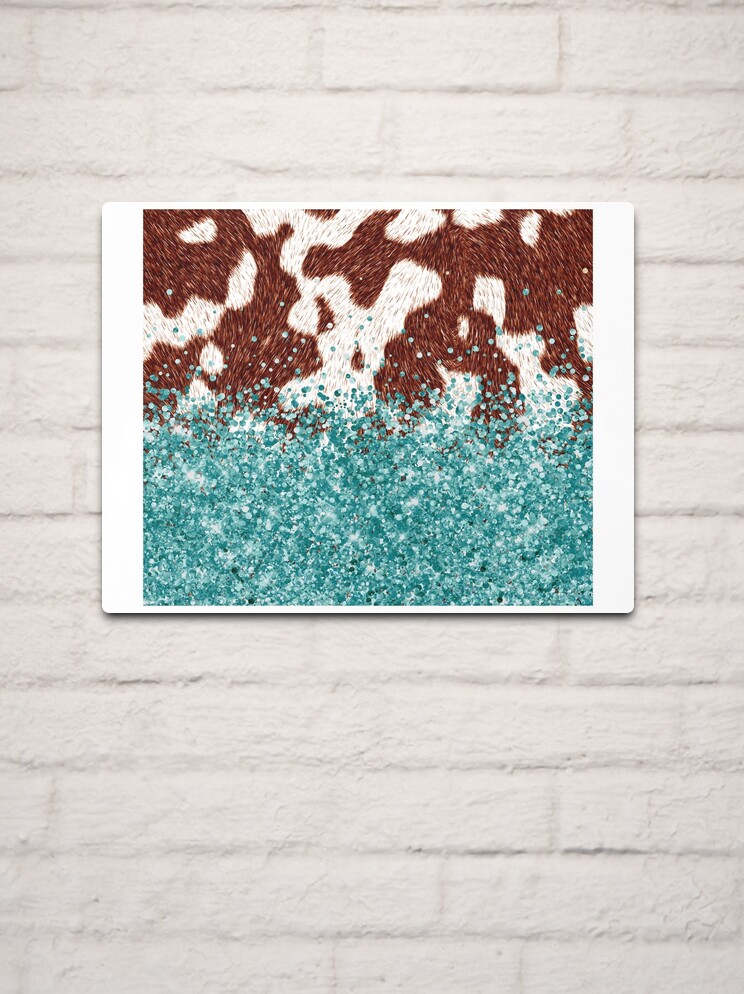The photograph depicts a section of a white-painted brick wall in portrait view. Mounted slightly above the midpoint of the wall is a landscape-oriented picture with an abstract design. This picture has a prominent white border, wider on the left and right sides compared to the top and bottom. The upper portion of the picture features a brown and white pattern resembling a cow hide, prominently showing curved lines and alternating patches of brown and white. The lower section transitions into a speckled, blue glitter-like texture with scattered turquoise and white points, creating a visual effect akin to water. This blend of natural and abstract elements is both intriguing and visually captivating, providing a stark contrast to the crisp white background of the wall.